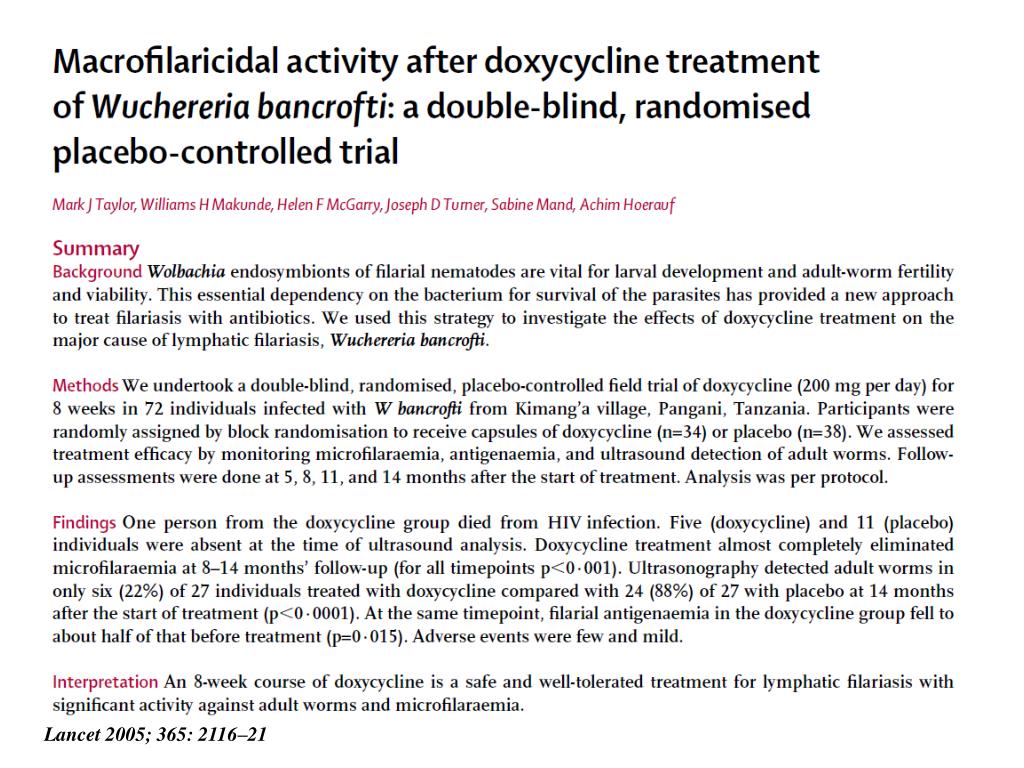"Macrophylaricidal Activity After Doxycycline Treatment of *Wuchereria Bancrofti*: A Double-Blind, Randomized, Placebo-Controlled Trial"

The article titled *"Macrophylaricidal Activity After Doxycycline Treatment of Wuchereria Bancrofti: A Double-Blind, Randomized, Placebo-Controlled Trial"* explores the impact of doxycycline on the nematode *Wuchereria Bancrofti*, which is the primary cause of lymphatic filariasis. The research involved leading experts in the field who conducted an in-depth study to understand how targeting the endosymbiotic bacteria essential for the parasites' survival could offer a novel treatment approach.

**Summary**

The background of this study hinges on the crucial relationship between filarial nematodes and their endosymbiotic bacteria, which are necessary for the nematodes' larval development, adult worm fertility, and overall viability. This dependency suggests that antibiotics like doxycycline could be effective in treating filariasis by disrupting this essential bacterial support system.

**Methods**

In a methodical approach, researchers conducted a double-blind, randomized, placebo-controlled field trial involving 72 individuals infected with *Wuchereria Bancrofti*. Participants received doxycycline treatment over an eight-week period, while another group received a placebo. This rigorous design aimed to eliminate bias and ensure reliable results.

**Findings**

The findings from this trial are detailed and demonstrate the potential efficacy of doxycycline in treating filariasis. Specific observations and measurements were taken to assess the impact on the nematodes, accounting for various biological markers and clinical outcomes.

**Interpretation**

Interpreting these results, the researchers draw significant conclusions about the therapeutic viability of targeting endosymbiotic bacteria to combat lymphatic filariasis. These insights may pave the way for new approaches to treatment and further understanding of the disease.

This comprehensive and meticulously conducted study offers promising data supporting the use of doxycycline as an innovative treatment for a condition that affects millions globally.